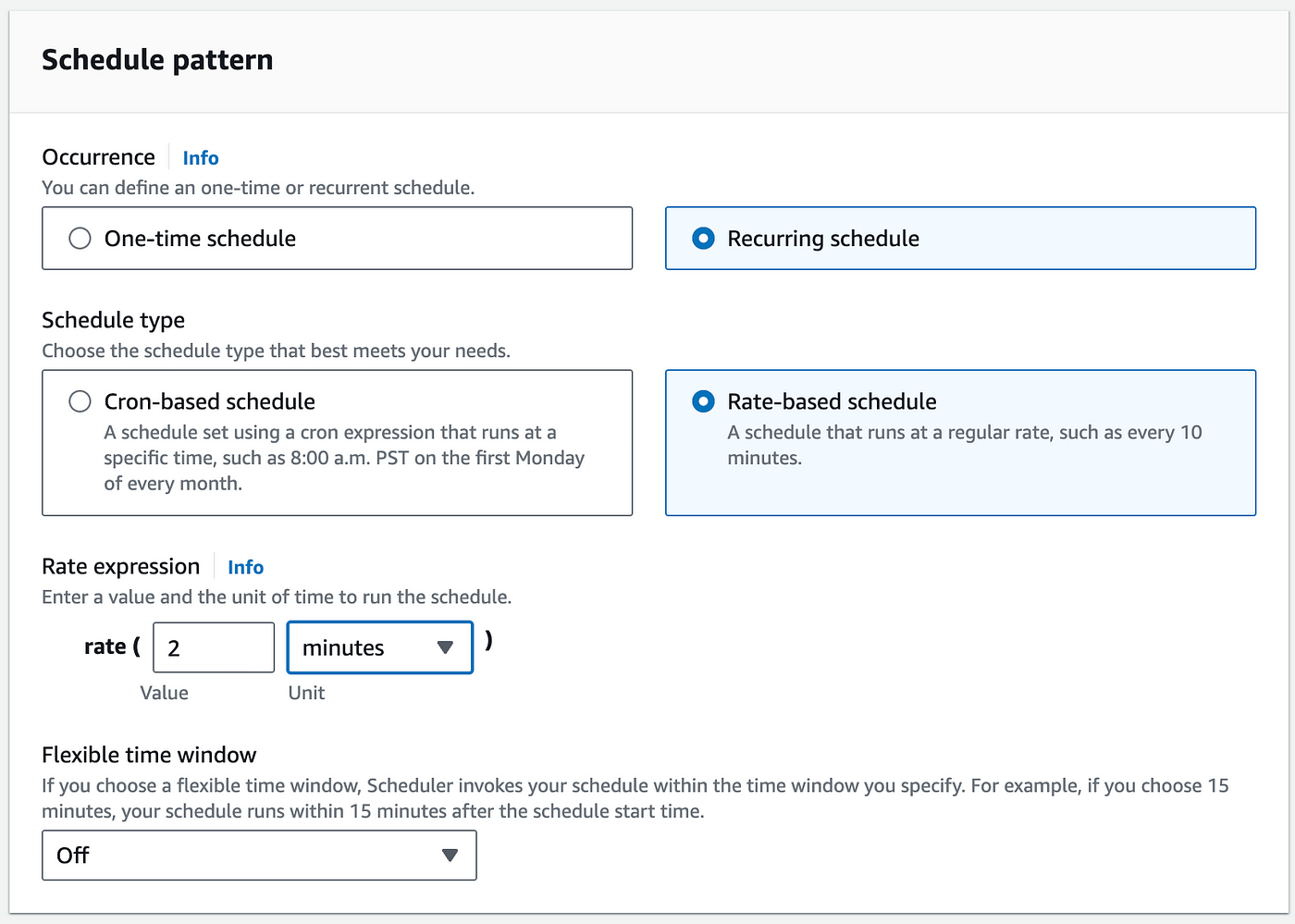The webpage appears to be designed for scheduling tasks. The interface features a clean, white background with neatly organized sections and distinct headers in bold black text. At the top of the page, the title reads "Schedule Pattern." Below this, there are two main sections: "Occurrence" and "Info," with the "Info" text displayed in blue.

The "Occurrence" section allows users to define schedules on either a one-time or recurring basis. On the left side, there is an option for a "One-time schedule" which is not selected. To the right, the "Recurring schedule" option is selected, indicated by a blue checkmark within a circle.

Further down, there is a "Schedule Type" section guiding users to choose between a "Cron-based schedule" and a "Rate-based schedule." The cron-based schedule option, located on the left, allows users to set a schedule using a cron expression for specific times, such as 8 a.m. PST on the first Monday of every month. The rate-based schedule option on the right, which is currently selected, enables scheduling at regular intervals, such as every 10 minutes. This selection is highlighted with a lit-up blue box.

Directly beneath this, the "Rate Expression" section prompts users to enter a value and time unit for the schedule frequency. The current settings specify a value of 2 and minutes as the time unit.

Lastly, the "Flexible Time Window" section, in black text, explains that selecting a flexible window allows the schedule to execute within a specified time frame after its start time. For instance, if a 15-minute window is chosen, the task will run within 15 minutes of the scheduled start time. Below this, there is a toggle to turn the flexible time window on or off.